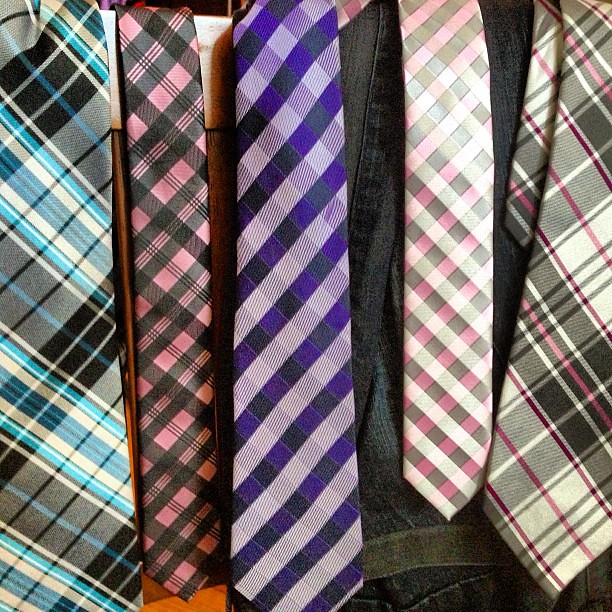In the photograph, we see a vibrant collection of neckties, all arranged horizontally from left to right and filling up most of the frame. They create a visually striking pattern with their varied plaid designs. On the leftmost side, there's a tie with a blue, black, and white plaid pattern. Next to it is another plaid tie in black and pink. The third tie from the left stands out with its bright violet, purple, black, and white plaid pattern. To its right, possibly draped over blue jeans, is a tie featuring pink, gray, and white plaid. On the far right, there's a larger diagonal plaid tie in white and black with pink pinstripes. The background shows a hint of wood and a suggestion of blue material, adding subtle context to the display without distracting from the ties. The overall composition is clean, focusing solely on the ties, which are typically worn with suits or for formal occasions, emphasizing their colors and patterns against a minimalist backdrop.